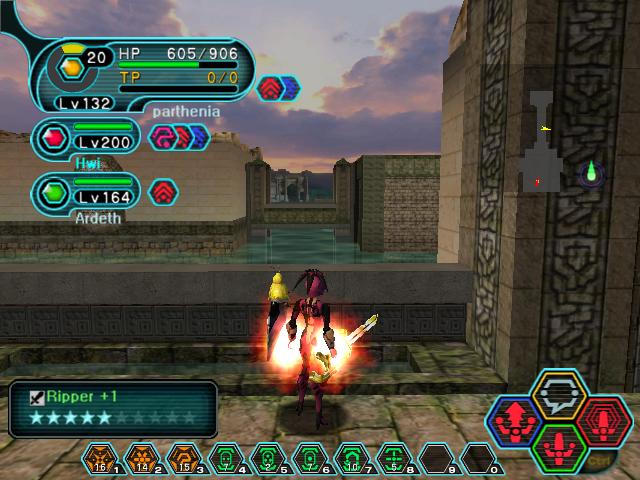This is a detailed screenshot from a fighter-type video game that blends realistic and blocky, Minecraft-like aesthetics. The background features a sunset sky streaked with blue, pink, and purple hues and adorned with fluffy clouds, contrasting with the realistic stone ground, walls, and aqueducts below. Central in the maze-like landscape stands a warrior character, illuminated by a bright white light, and dressed in a purple costume with a helmet that has hair sticking out, carrying a sword and shield, and bearing a pistol on their thigh. Another smaller, yellow character is also present near them. The player's name, "RipperPlusOne," is listed in the lower-left corner. The screen is filled with information indicators; the top left corner shows fighting and status indicators, while an overhead map showing the player's location is displayed in the upper right. Along the bottom of the screen, various icons represent levels of achievement and accessible tools, forming a cache storage area.